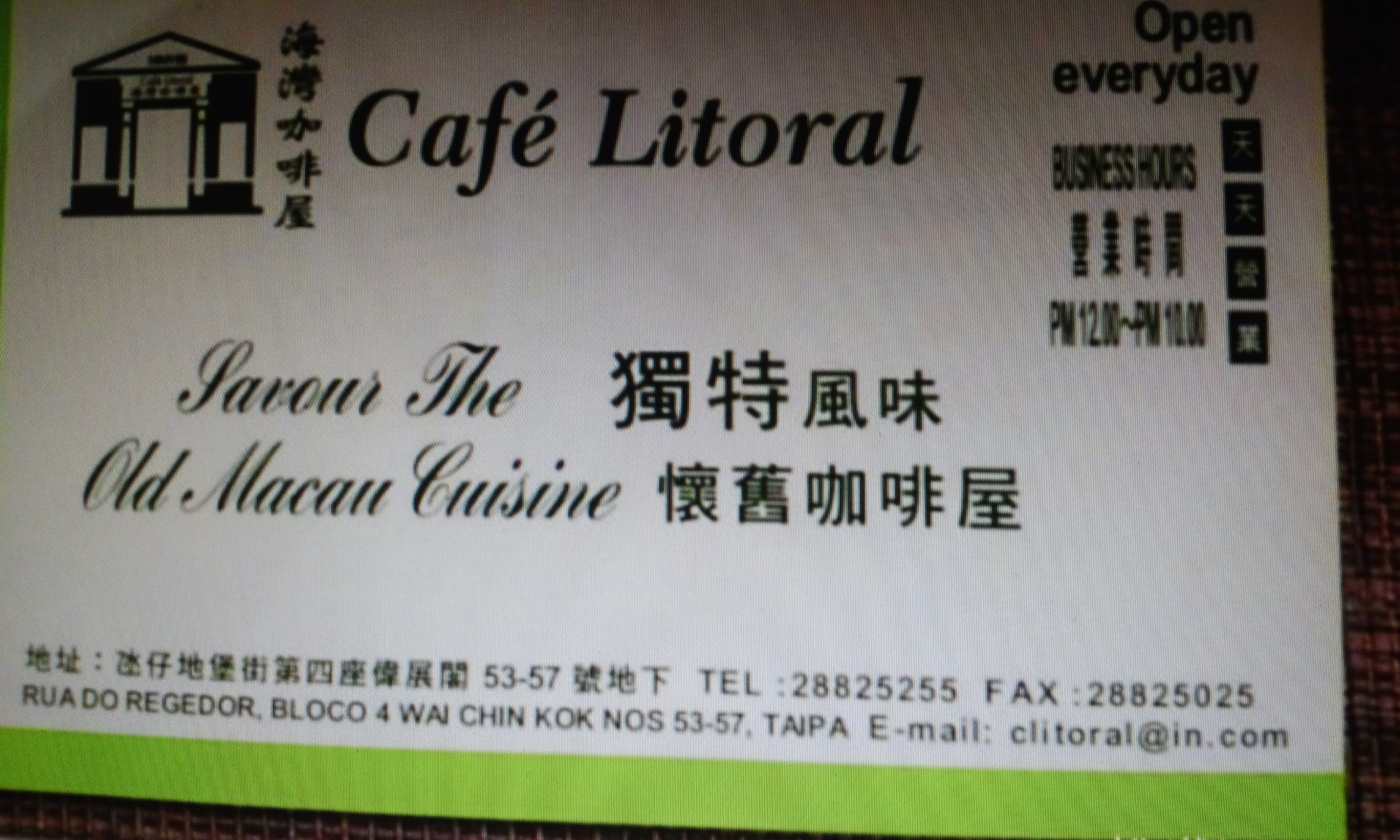The image showcases a white background with a lime green border at the bottom. At the top left corner, there is an icon that resembles a small house or shelter, alongside vertically arranged Chinese characters. To the right, the text "Café Litoral" is displayed in black font, with an accent above the 'E'. The top right corner announces "Open Every Day" followed by "Business Hours," likely in Chinese, and then in English, "P.M. 12 - P.M. 10," indicating unclear operating hours. Centered on the image are the words "Savor the Old Macau Cuisine," with a probable Chinese translation beside it. The bottom part of the image contains extensive Chinese text, contact information, and address details. It lists "53-57," phone number "28825255," fax "28825025," and the address "Rua do Regedor Bloco 4, Taipa." Lastly, an email address, "cafe_litoral@in.com," is provided.